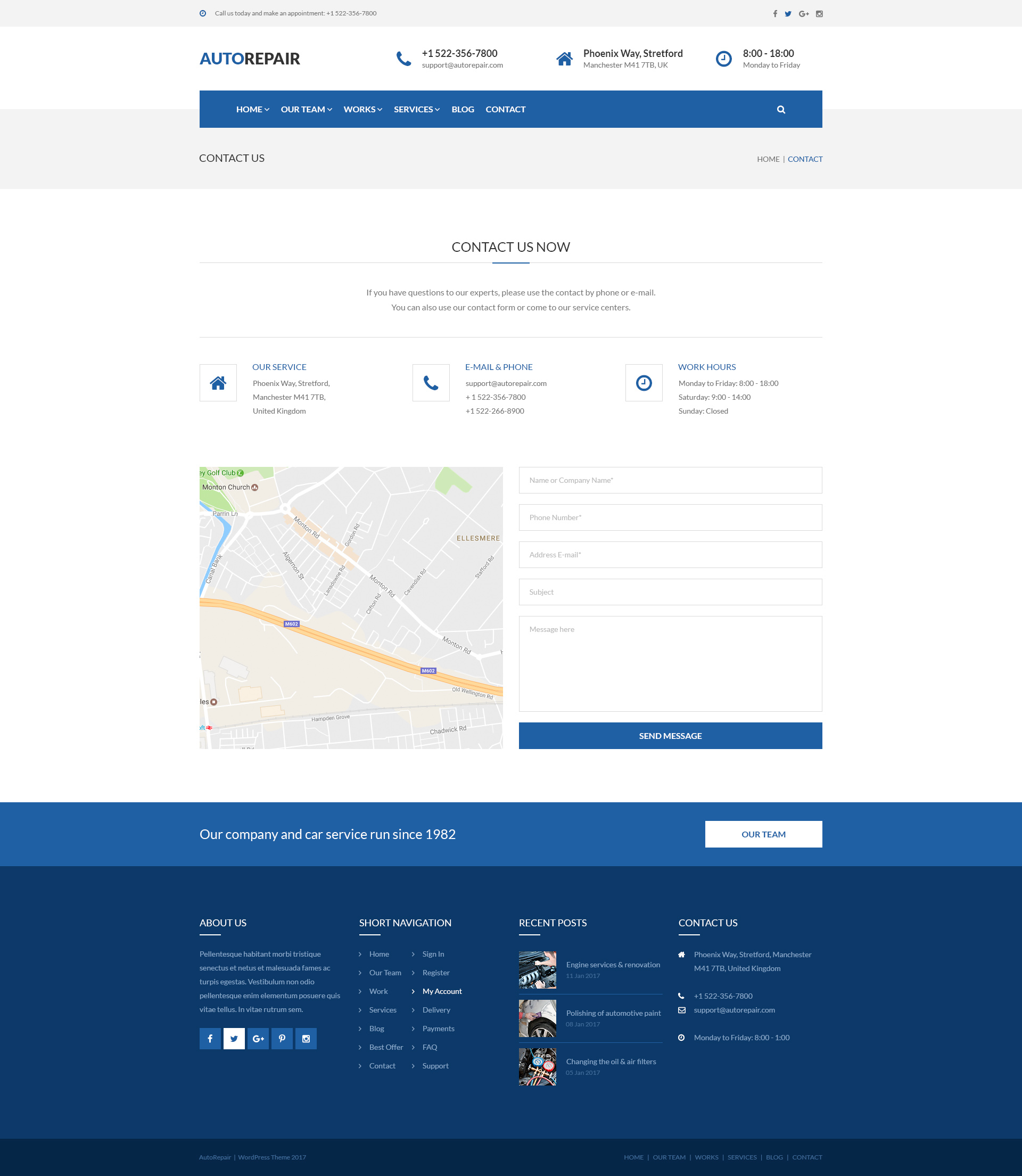**Contact Us for Professional Auto Repair Services**

This digital image provides comprehensive contact information and details about a reputable auto repair service. 

- **Phone Number**: +1 522-356-7800
- **Email Address**: support@autorepair.com
- **Physical Address**: Phoenix Way, Stratford, Manchester, M41 7TB, UK
- **Operating Hours**: Monday to Friday, from 08:00 to 18:00
- **Social Media**: Facebook and Twitter logos are displayed
- **Contact Information**: You can reach out to our experts via phone or email, or use our contact form available on our website. Alternatively, feel free to visit our service centers.

The image also includes a map for easy navigation to the service center. 

**About Us**: Our company has been providing top-notch car repair services since 1982.